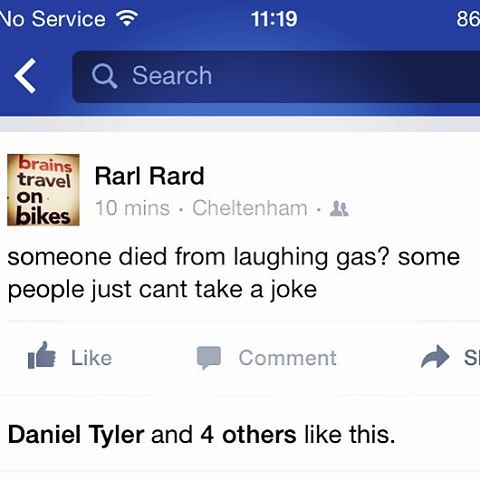This image is a detailed screenshot from an iPhone displaying a Facebook post. At the top, it indicates "No Service" with the time shown as 11:19 in the center and an 86% battery level on the right. Below this, a thicker blue dashboard features a back arrow and a search button. The central content is a post by Raul Rod from 10 minutes ago in Shelterham, humorously captioned with his profile picture showing "brains travel on bikes." His post reads, "Someone died from laughing gas. Some people just can't take a joke," and has received likes from Daniel Tyler and four others.